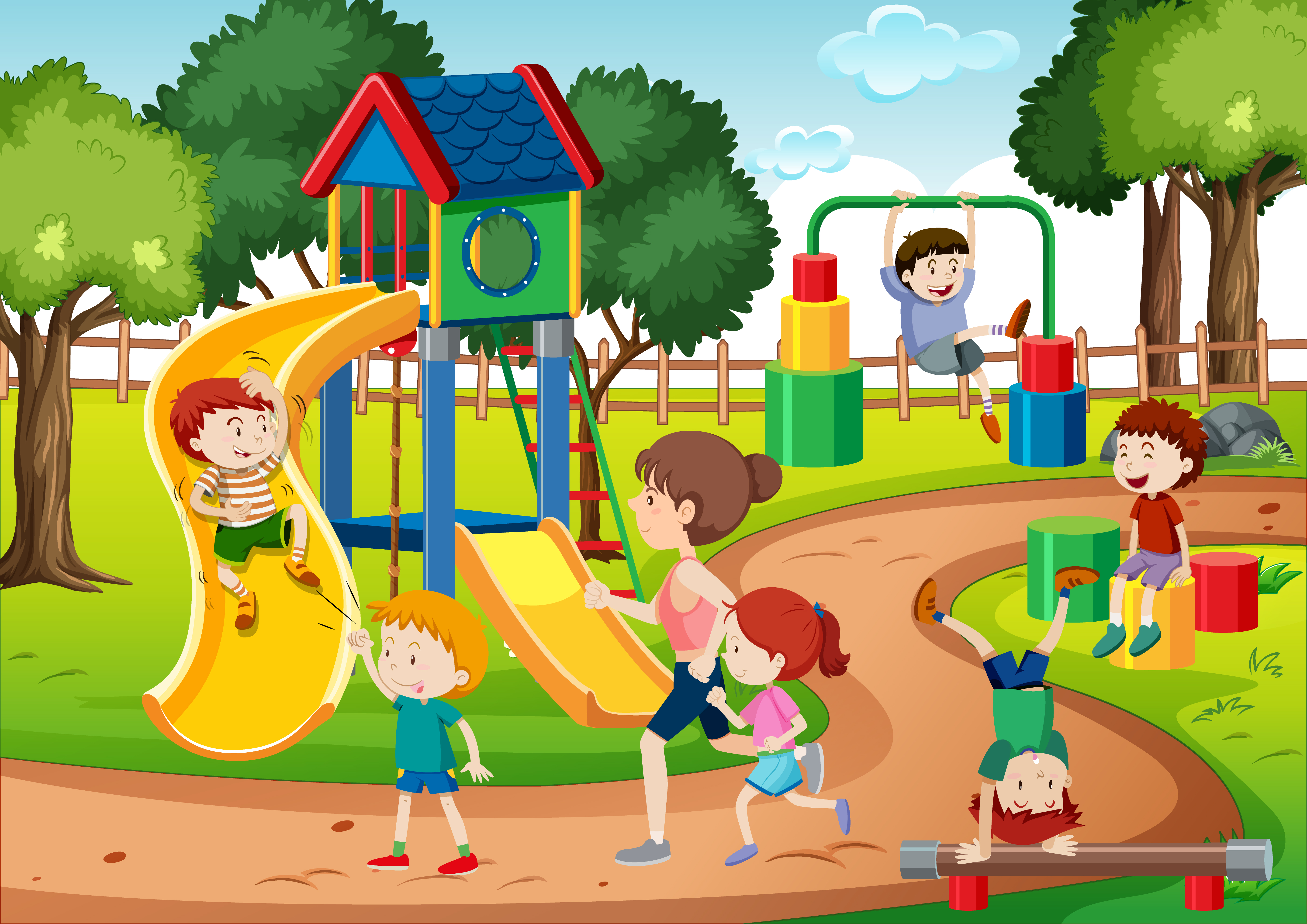This vibrant and detailed vector illustration depicts a lively playground scene filled with activity and colorful elements. At the heart of the playground, there is a central tower adorned with a blue roof and red accents, featuring a yellow slide with a child joyfully sliding down. The tower also includes a ladder, a little window, and an additional smaller yellow slide at its base. Surrounding the central tower, numerous children can be seen engaging in various activities: some are running along a snaking path that curves from the middle to the bottom left of the image, others are playing on a balance beam, and still others are hanging from playground equipment. A child is even standing on a log with some seating nearby, and another is performing a handstand. 

The playground is enclosed by a wooden fence, and the lush surroundings are dotted with trees exhibiting different shades of green leaves and brown trunks, set against a backdrop of a clear blue sky with a few scattered clouds. Towards the right side of the image, a mother jogs alongside her child, adding to the energetic atmosphere. The rich color palette features greens, yellows, reds, browns, blues, and grays, contributing to the overall cheerful and dynamic vibe of the playground. This digital rendering evokes a sense of joy and playfulness, reminiscent of illustrations from children's books or animated TV shows like "Caillou" or Disney cartoons.